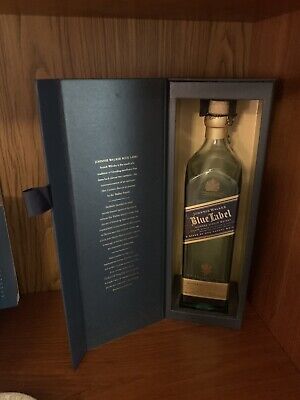This is a photorealistic image of a rectangular wooden cabinet, showcasing an open box of Johnny Walker Blue Label whiskey. The box, which is predominantly black with gold interiors, features a flap with a column of intricate, yet unreadable, gold text. The standout item is the clear glass bottle of whiskey, prominently displayed within the box. The bottle is adorned with a distinctive blue label inscribed with "Blue Label" in white text, complemented by gold borders and a gold cap. Additionally, just peeking out from the frame to the left is another similar blue box, suggesting the presence of more bottles. The entire setup exudes a sense of sophistication and selective presentation, highlighting the premium nature of the product.